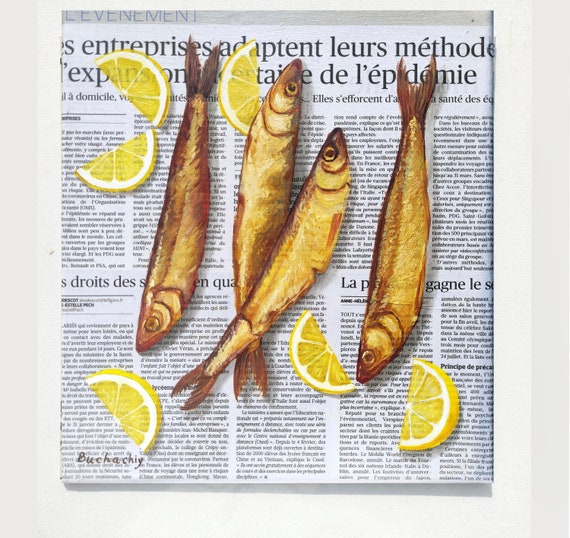In the center of this image, a square-shaped piece of folded newspaper, in a bluish-gray tone with black text, showcases the headline "Enterprises Adaptant Lures Methods," suggesting it might be in French. Placed on this newspaper are four whole, golden-brown fish, reminiscent of sardines. The fish, with heads and tails intact but fins removed, are arranged with the ones on the sides facing downwards and the two in the center crossed and facing upwards. Scattered among them are several yellow lemon slices, some partially transparent, contributing to the arrangement. The newspaper rests on a background with medium and light gray borders, creating a simple yet striking composition against the off-white backdrop. The newspaper’s text includes black headlines and various paragraphs, adding a textual element to the otherwise culinary display.